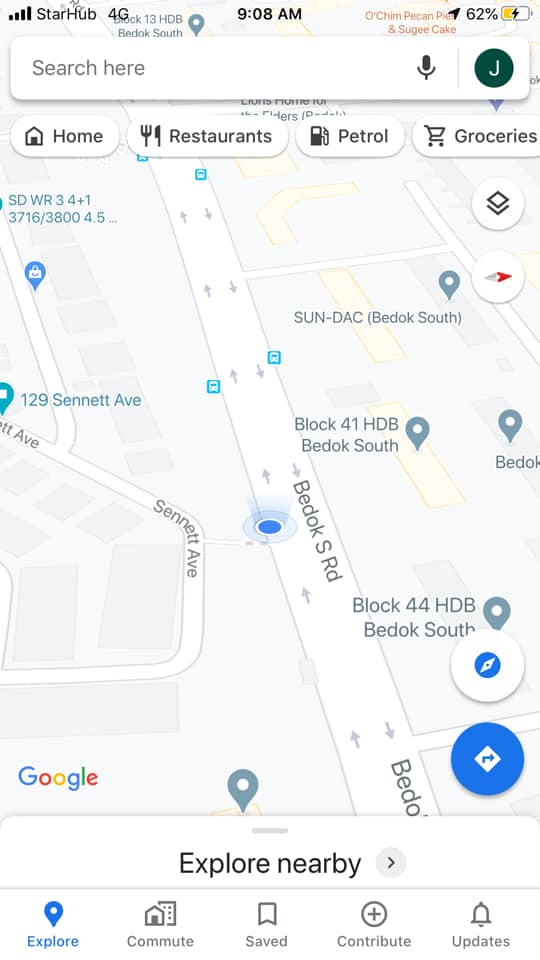This image features a series of mobile device screenshots, prominently showcasing various interface elements. The network provider displayed is Starhub, but the network signal bars are barely visible. The device clock indicates the time as 9:08 AM, and the battery level, positioned in the top right corner, stands at 62%. Lower on the screen, a search box is present, with example locations such as Bedok S Road, Block 44 HDB, and Sundark entered. Additionally, several category tabs are visible, labeled as Explore, Commute, Save, Contribute, and Update.